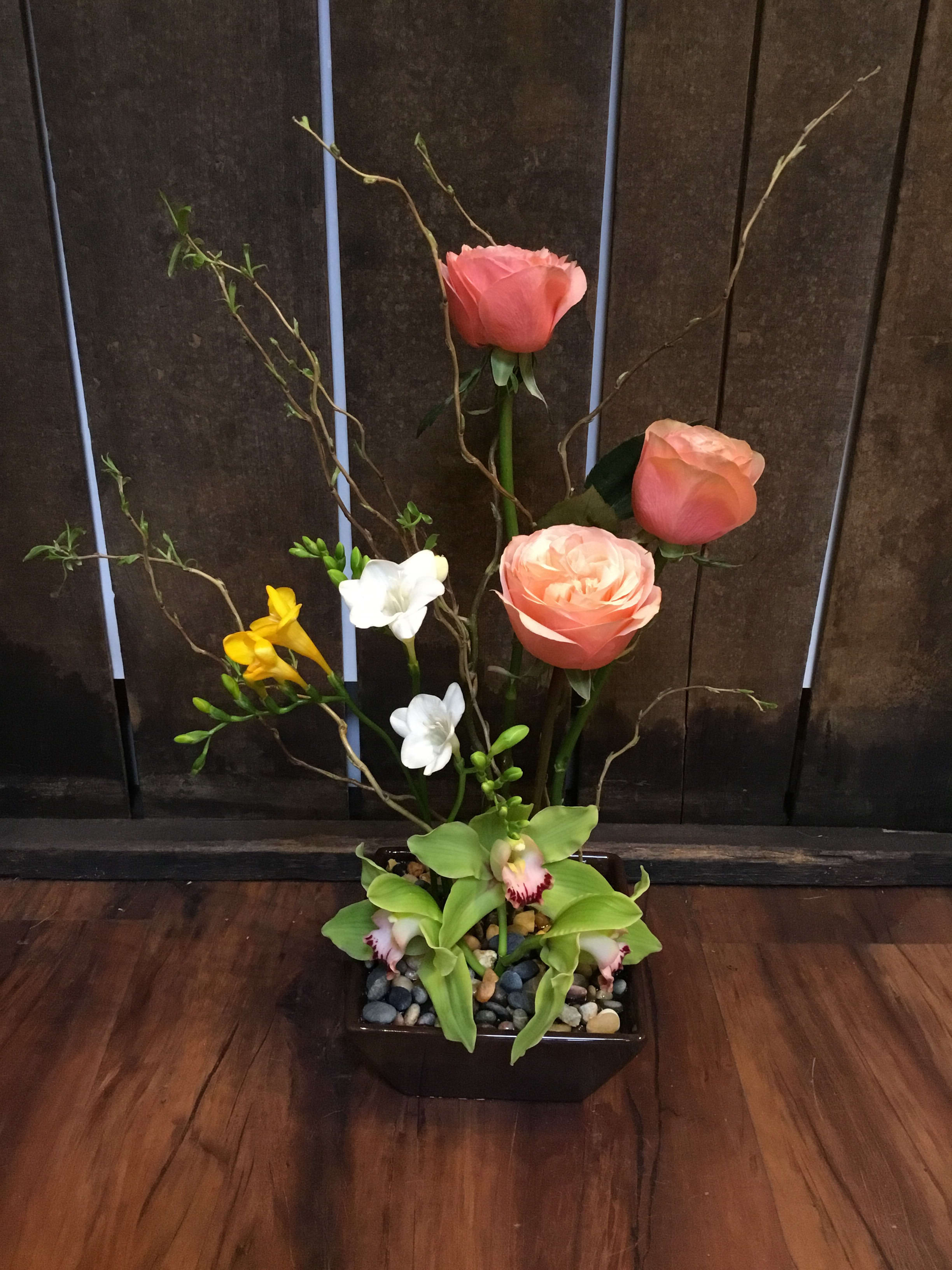The photograph displays a carefully arranged floral bouquet set on a polished wooden floor with a medium brown and dark wood grain pattern. The backdrop is a darker wooden structure, potentially decorative fencing or an aged wooden wall. The bouquet sits in a low, dark marble vase filled with multicolored pebbles—gray, white, and yellow—and bright green leaves. The floral arrangement itself is colorful and detailed: on the right, three pink roses are prominently positioned, while to the left are white flowers resembling lilies and further left, some yellow daffodils are yet to fully bloom. The green stems and leaves not only fill the base but also extend past the flowers, adding a sense of natural growth and vibrancy.